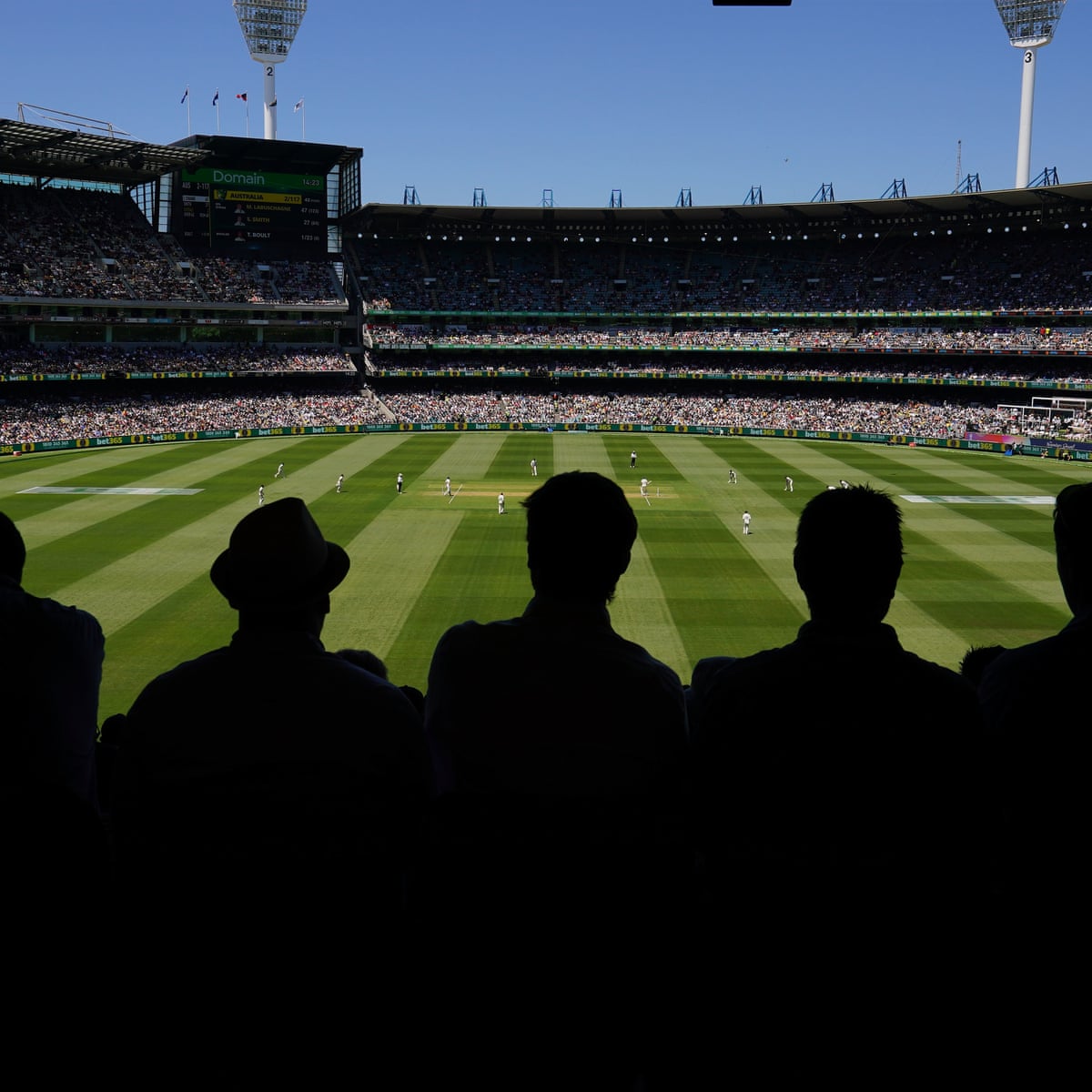This photograph captures a vibrant and packed stadium during a sunny day with a clear, Carolina blue sky. The large, circular stadium is filled with spectators from the foreground to the farthest reaches on the other side, emphasizing the excitement of the event. In the foreground, five men are shown in shadowed silhouette, one of whom is wearing a hat, as they intently watch the game being played on the field. The lush green grass of the field is neatly striped in alternating dark and light green, adding to the scene's meticulous appearance. Although there is some confusion about whether it's a baseball or cricket match, the essence of a well-manicured sports field is clear. Above the scoreboard, which reads "domain" or possibly "Australia," four flags flutter in the breeze, adding to the grandeur of the setting. The photograph encapsulates a perfect day for sports, with detailed visuals from the shadows of the spectators to the packed stands and the pristine condition of the playing field.